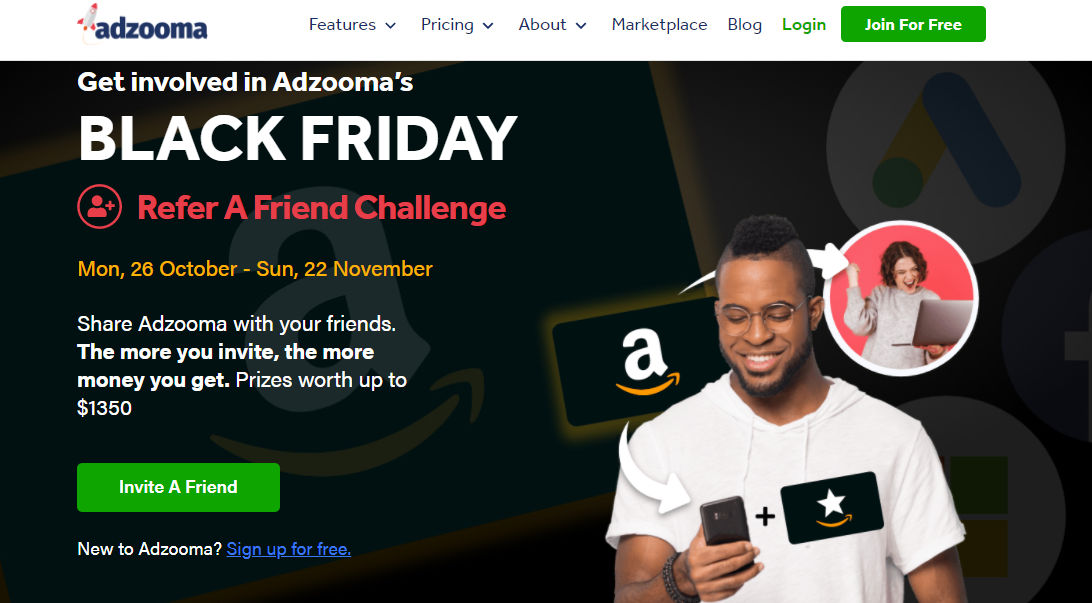This image, sourced from the Adzooma website, features a detailed and visually segmented layout promoting a special event. At the top of the webpage, there is a navigational menu with clickable areas labeled as: Features, Pricing, About, Marketplace, Blog, Login, and Join for Free. Notably, 'Login' is highlighted in green font, while 'Join for Free' appears in white text within a prominent green box.

Progressing down the page, a black background hosts a promotional banner for Adzooma's "Black Friday Refer a Friend Challenge" outlined in attention-grabbing red text. Below this, a timeline is displayed in orange text with the event spanning from Monday, October 26 to Sunday, November 22.

Further down, a white text block encourages users to "Share Adzooma with Your Friends," emphasizing that increased invitations correlate with higher monetary rewards, potentially reaching up to $1,350. Adjacent to this message is a green 'Invite a Friend' button.

Beneath the invite option, a white text prompt for newcomers reads "New to Adzooma? Sign Up for Free," with 'Sign Up for Free' distinguished in blue font.

The image also includes a photograph featuring a man holding a cell phone. He stands against an Amazon 'swoosh' backdrop, wearing a shirt branded with the Amazon logo, alongside an image of a girl, further emphasizing the collaborative and social nature of Adzooma's campaign.